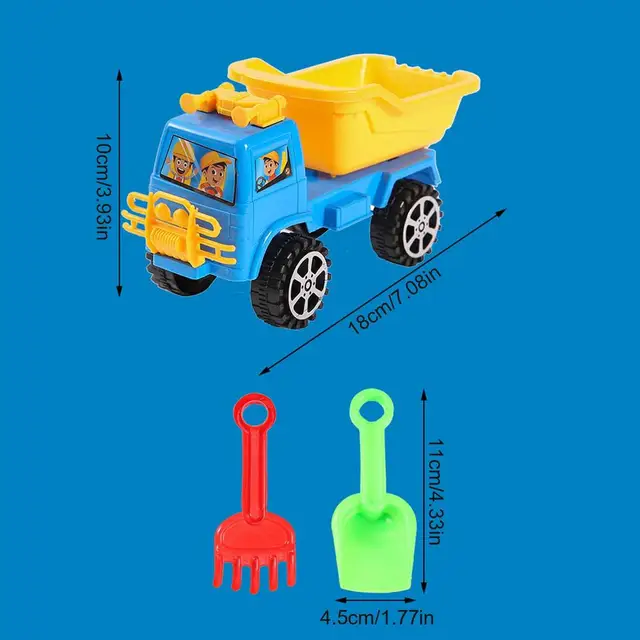The product photograph features a set of vibrant children's toys displayed against a solid blue background, ideal for commercial use in an online catalog or shop. Prominently positioned at the top of the image is a detailed toy dump truck. The truck boasts a striking blue body with a yellow bumper on the front and a distinctive yellow horn-shaped object on the roof. It features a yellow plastic bucket on the back, four large and rugged black plastic tires, and windows adorned with stickers depicting two young boys in construction outfits driving the truck. The dimensions are clearly indicated with arrows; the truck measures 10 centimeters (3.93 inches) in height and 18 centimeters (7.08 inches) in length.

Below the truck sits a plastic green shovel and a red plastic rake. Both tools are presented with their measurements, showcasing their sizes for potential buyers: the shovel stands 11 centimeters (4.3 inches) tall and 4.5 centimeters (1.77 inches) wide. Similarly, the rake has comparable dimensions and distinct color coding for easy recognition. Each handle features a hole at the top for convenient hanging or storage. With precise dimensions and detailed descriptions, this photograph offers a comprehensive view of the product, perfect for online retail environments.